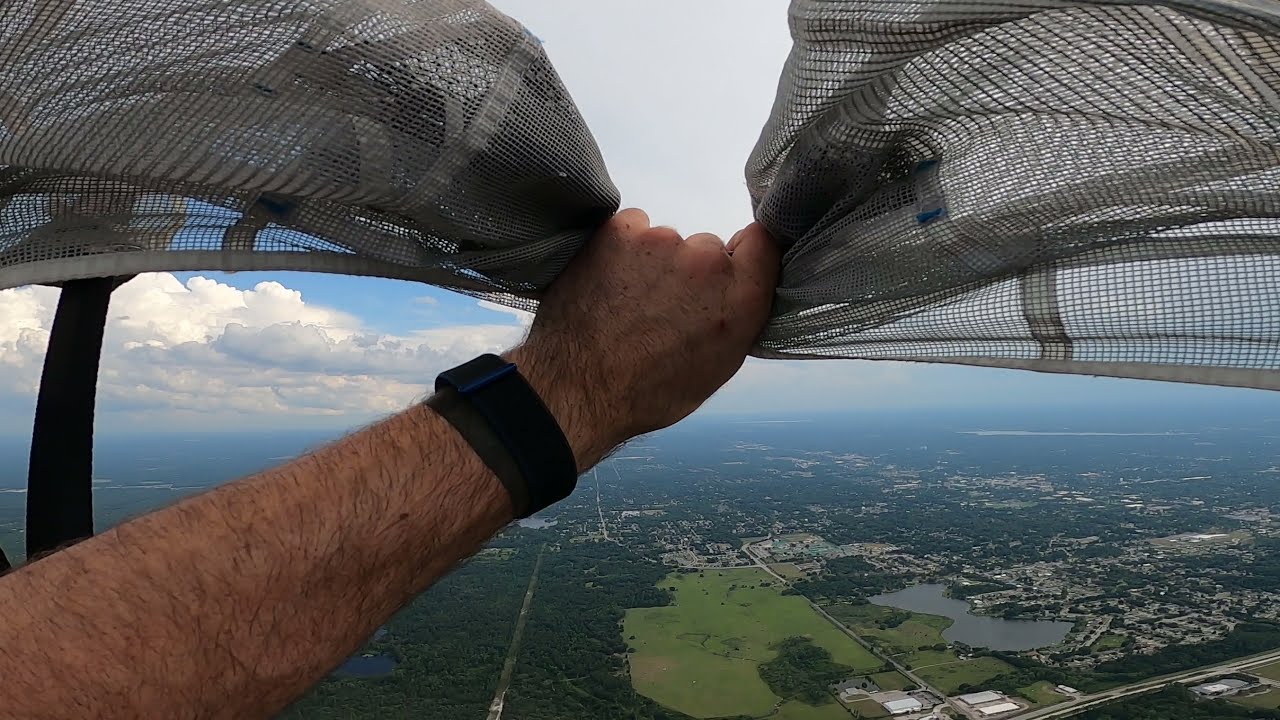The photo captures a scene high up in the sky, akin to skydiving or hang gliding altitude. The background reveals a panoramic view of Earth below, featuring vast green fields, clusters of trees, specks of small white buildings, and bodies of water. The horizon is partially obscured by haze, making ground details faint. Above, the sky is a vibrant blue, adorned with large, fluffy clouds. Dominating the foreground is a man's left arm, notably hairy, extending from the lower left corner of the image. He is wearing a black wristband and gripping a piece of gray mesh netting, which he appears to be holding or pinching tightly so that it bunches at the center. There is a black pole visible on the left side, which seems to partially support the netting. The entire composition provides a thrilling sense of altitude and adventure.